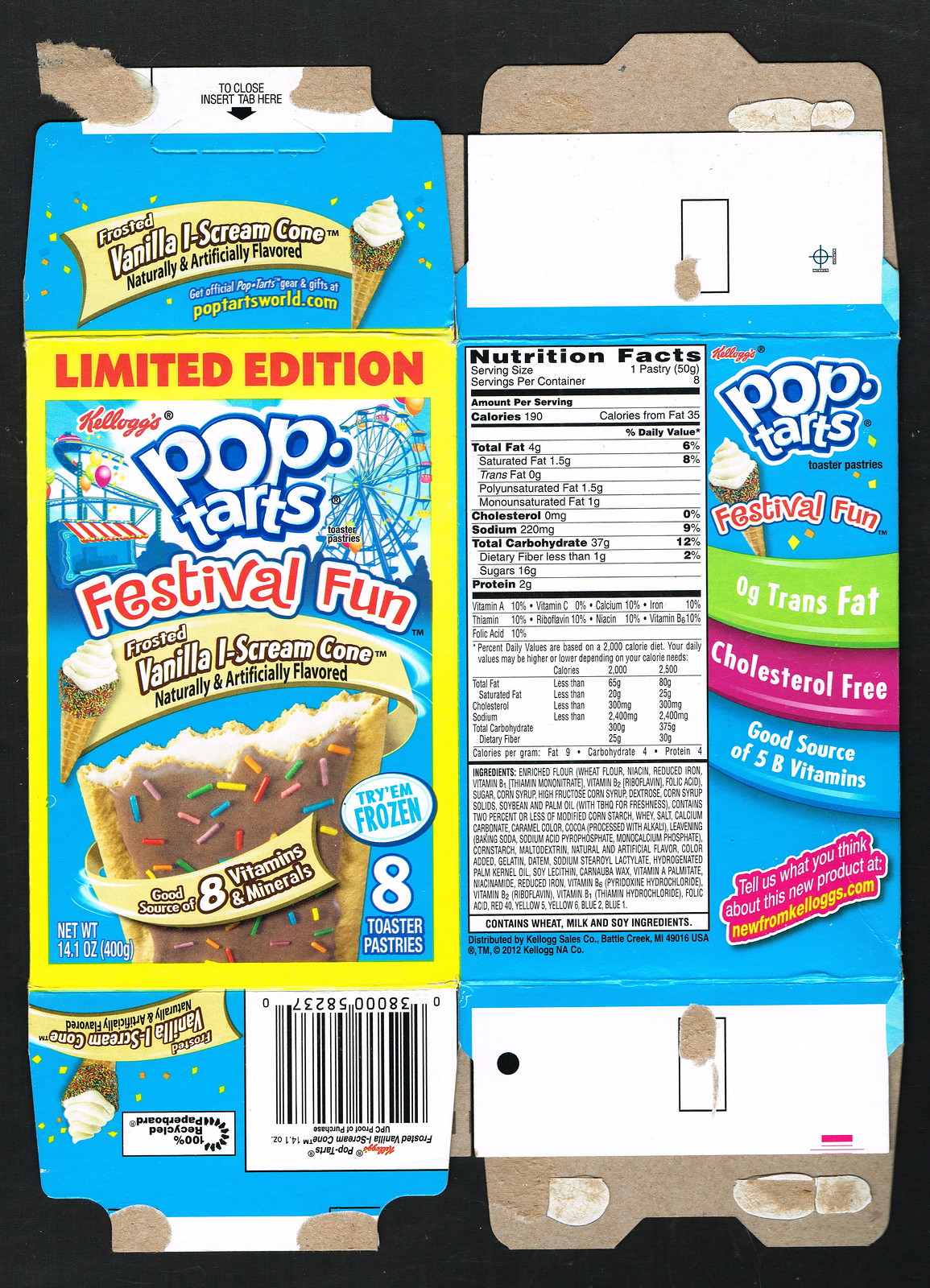This image features a flattened cardboard Pop-Tarts box set against a black background. The box, captured in its entirety and laying flat, is primarily colored in white and sky blue hues. On the left portion of the box, bold letters announce it as a "Limited Edition" product: "Pop-Tarts Festival Fun Frosted Vanilla Ice Cream Cone". The flavor, described as "Naturally and Artificially Flavored," is visually depicted with an image of a partially eaten Pop-Tart. The Pop-Tart has brown frosting, adorned with multicolored sprinkles, and a white interior. Behind this label, there is an illustrated background featuring an amusement park, adding a whimsical touch to the packaging.

To the right of this playful label, the detailed nutrition facts are displayed. The facts highlight key health information, including "Zero grams of trans fat," "Cholesterol free," and "A good source of 5 B Vitamins." The flattened state of the box reveals additional aspects: the folded flaps of the cardboard, with visible glue remnants, offer a glimpse into its manufacturing process. Overall, the box's vibrant design and detailed information make it visually engaging and informative.